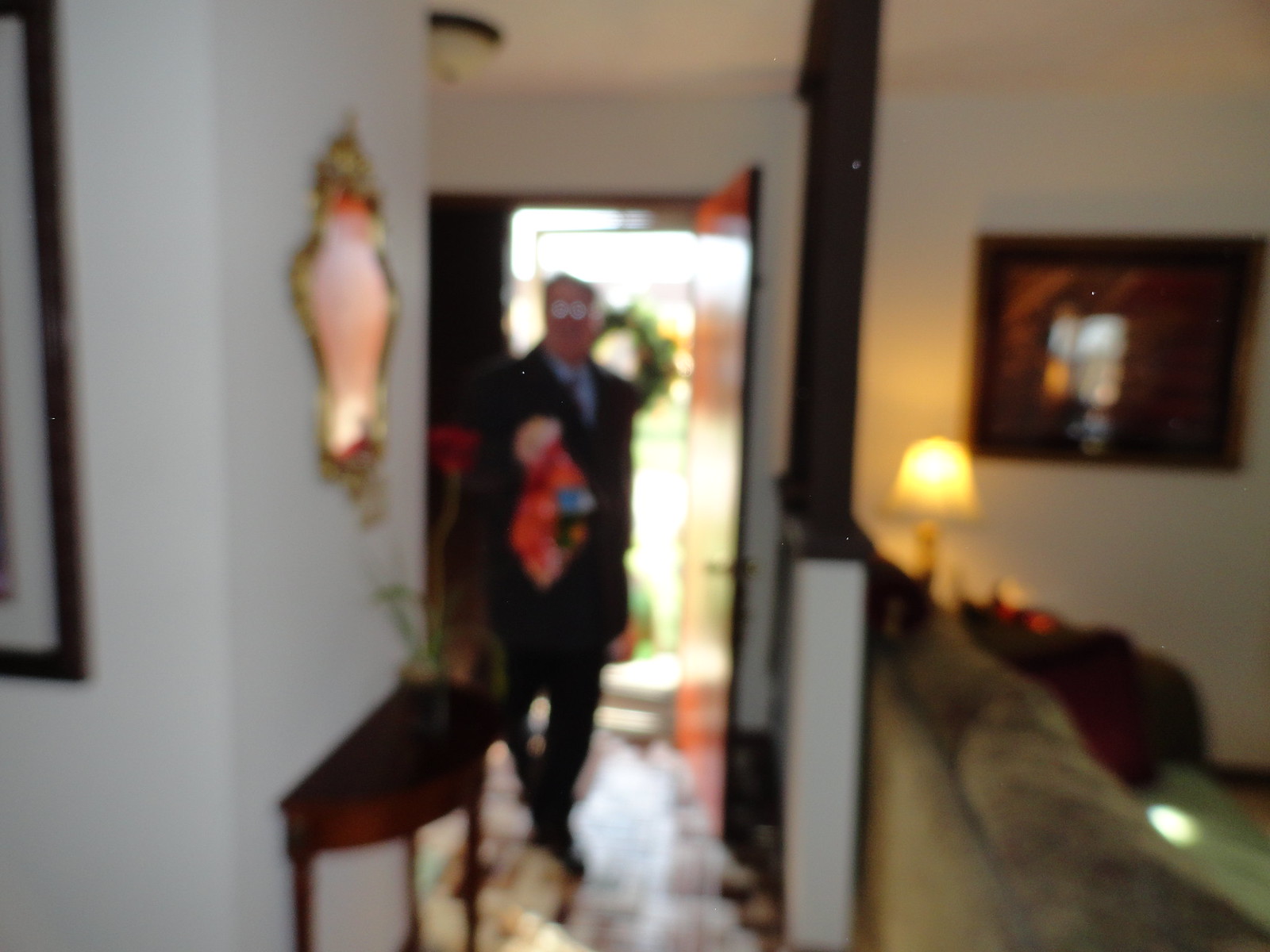In this very blurry image, an older man walks into a house through a front door that's slightly ajar, revealing a screen door adorned with a holiday wreath. The man, clad in a black suit, black shoes, and glasses, extends his right hand holding something red and blue, possibly a gift. His eyes appear to shine brightly, though the details are indistinct due to the blurriness. The entryway features a dark brown table adorned with a green-stemmed, red-flowered plant in a black pot, positioned beneath a unique, vintage gilded gold mirror. To the man's left, a cozy living room or family room is partially visible, showcasing a big suede couch, a lit lamp, and a piece of art on the wall.